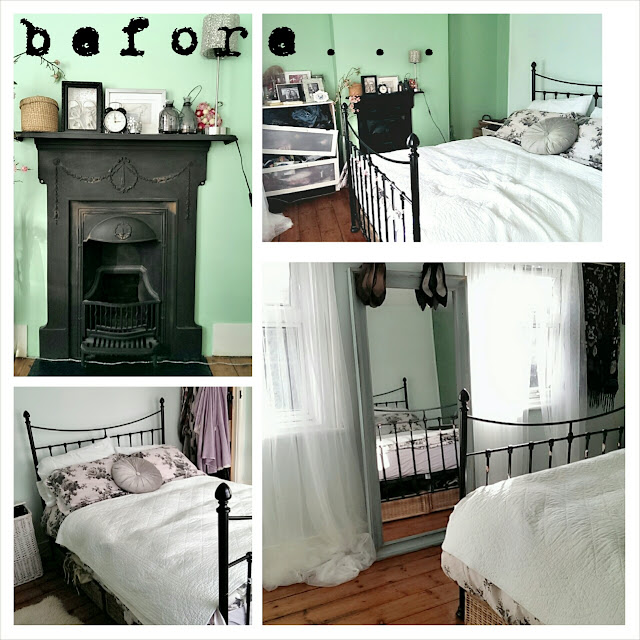The image is a collage of four photographs depicting a single bedroom in various stages of disarray and organization, collectively labeled "before..." in a scratchy font at the top. 

In the upper left photograph, there is a tall, slender black fireplace adorned with numerous items including a basket, a black alarm clock, two picture frames, a silver ornament, assorted jars, and a lamp, all set against a lime green wall. The upper right image reveals the same room, showing a bed with a black metal frame, white sheets, and gray pillows. Alongside the bed, there's a worn-out dresser laden with picture frames and other miscellaneous clutter.

The bottom left picture offers another perspective of the bed, now showcasing floral-decorated pink pillows and some purple clothes hanging nearby. The wall appears duller and more grayish in this shot. The bottom right photograph, the largest in the collage, displays a more organized view with neat white translucent drapes over two windows, a tall full-length mirror balancing between them, and shoes hanging from the mirror's frame. The same bed from previous photos sits neatly tidied, set against bright orange hardwood floors, completing the room's transformation.